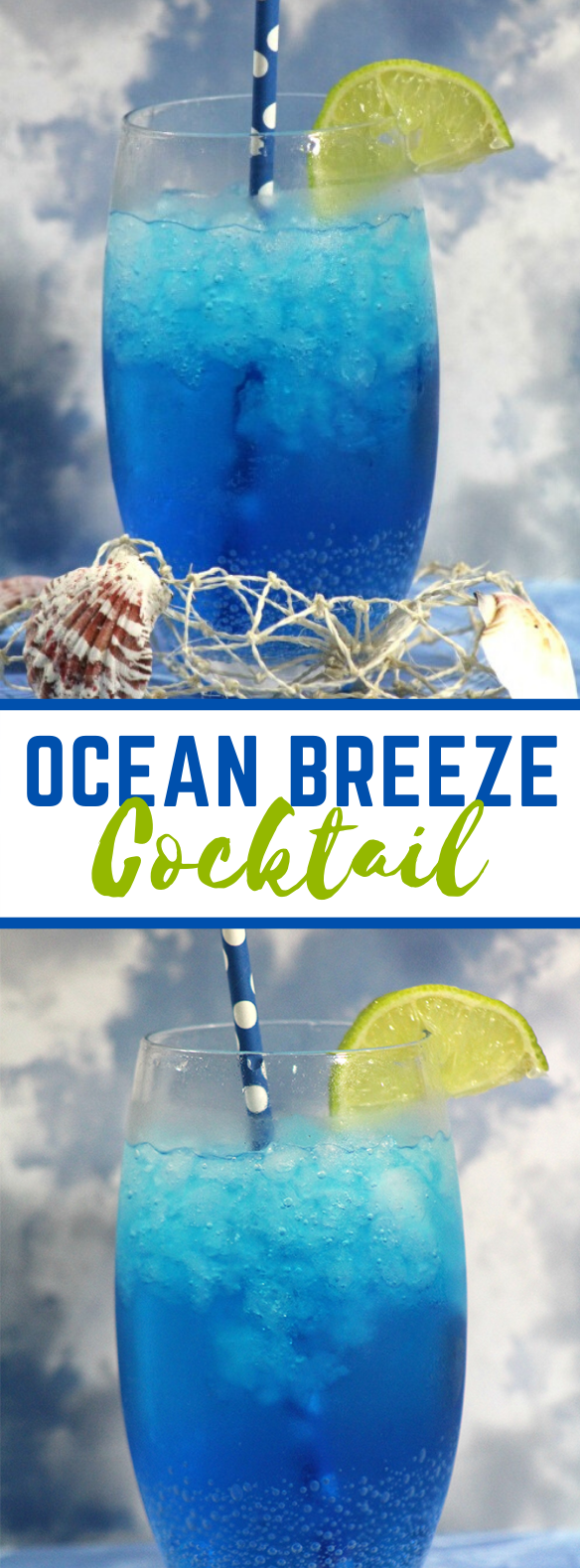This image captures a smartphone screenshot displaying two stacked photographs. Each photograph features a glass filled with a vibrant blue liquid, ice cubes, and a straw. A wedge of lime is elegantly attached to the rim of the glass. In the background of both images, the sky is adorned with fluffy clouds, creating a serene atmosphere. The foreground showcases an array of seashells scattered on the surface supporting the glass, adding a beachy vibe to the composition. Separating the two photographs is a white strip with the phrase "OCEAN BREEZE" written in bold blue capital letters, followed by the word "COCKTAIL" in green lettering directly below.